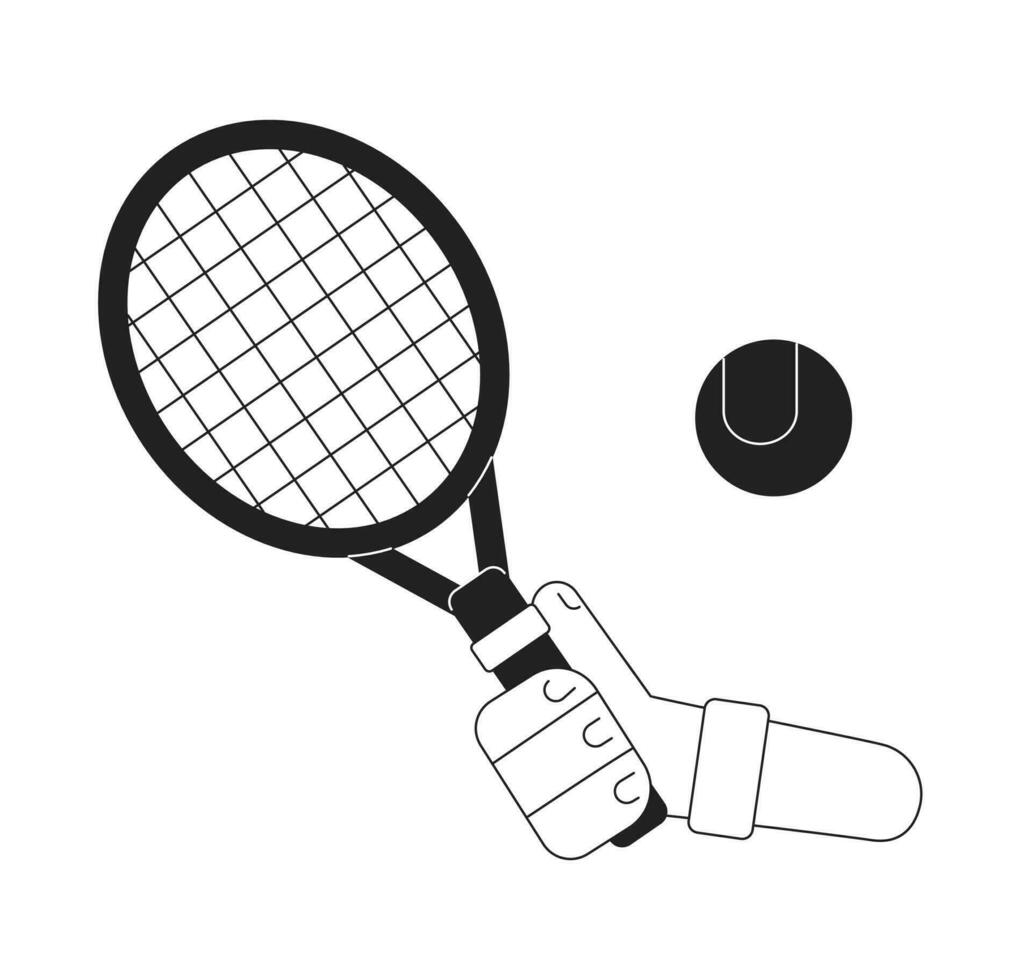A simplistic, black-and-white drawing showcases a hand with three fingers and a thumb, each detailed with fingernails, grasping a short-handled racket. The racket, predominantly black with a white stripe near the handle, has a simplified net pattern. The handle appears notably short, potentially indicating it could be a racket ball racket rather than a traditional tennis racket. To the side of the hand is a black tennis ball featuring a distinctive U-shaped white line, resembling a half-cut cylinder. The hand, outlined in black and filled mostly in white, is depicted emerging from a long-sleeved shirt, with the cuff visible. The overall minimalist style of the drawing suggests it could be an instructional or promotional poster for tennis.